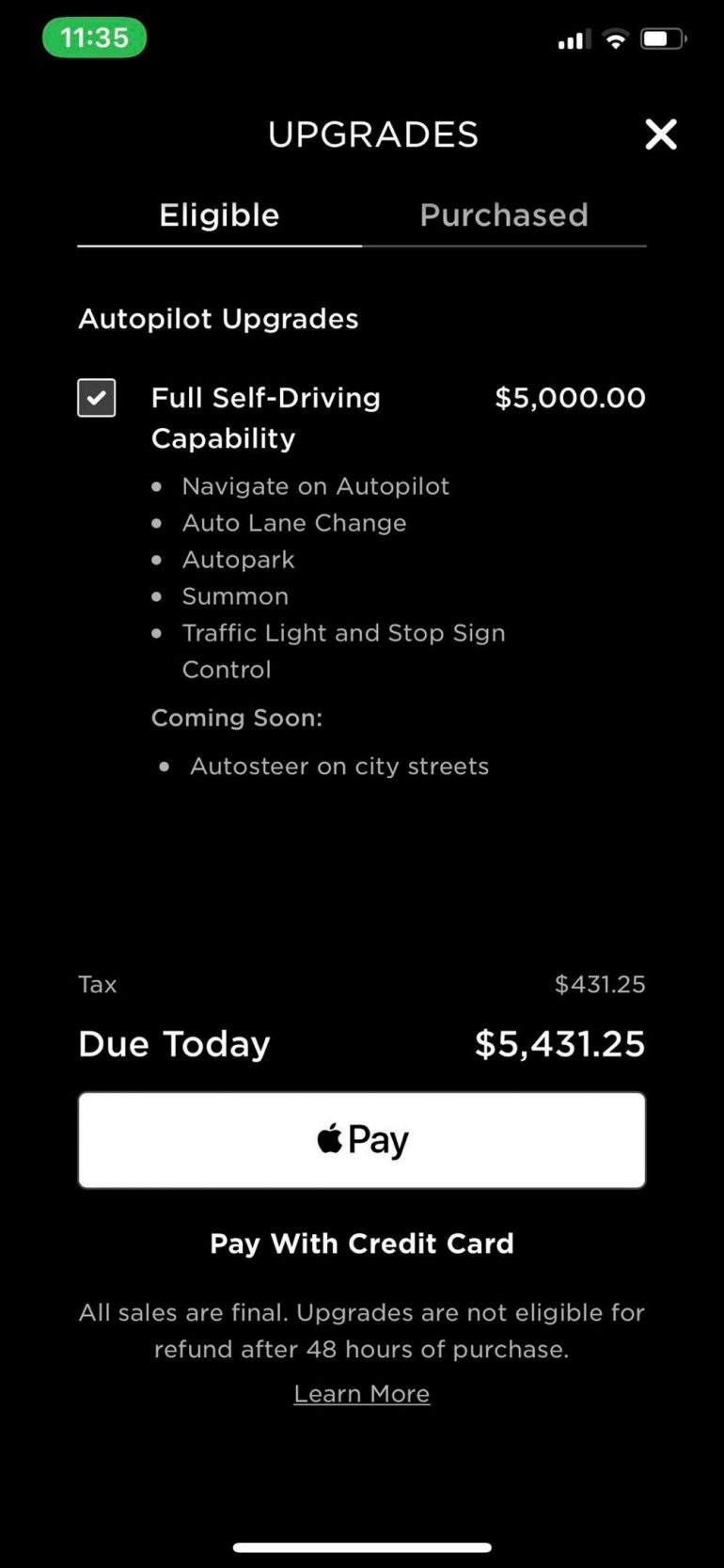The screenshot displays a section of a mobile application. At the very top, the time is shown as 11:35, framed by a green outline indicative of an ongoing call. Below the time, the word "Upgrades" is prominently featured, with an "X" button to the right for closing the window.

The interface is divided into two tabs: "Eligible" and "Purchased." The "Eligible" tab is currently selected. Within this tab, details for "Autopilot Upgrades" are listed, specifically highlighting the "Full Self-Driving Capability" upgrade priced at $5,000. The description provides a comprehensive list of features including "Navigate on Autopilot," "Auto Lane Change," "Auto Park," "Summon," and "Traffic Light and Stop Sign Control." An upcoming feature, "Auto Steer on City Streets," is also mentioned.

Additional financial details are displayed: a tax of $431.25, making the total amount due today $5,431.25. Below this, there are payment options including an Apple Pay button and an alternative to "Pay with Credit Card." A disclaimer notes that "All sales are final," and upgrades are non-refundable after 48 hours of purchase. Lastly, there is a "Learn More" button for further information.